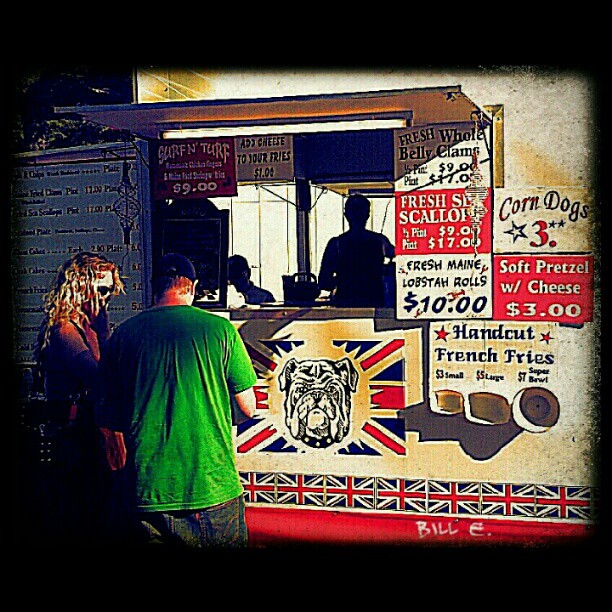The image depicts a man and a woman at a food truck named "Surf and Turf" that offers takeout. The man is wearing a green shirt, blue jeans, and a hat, while the woman has long blonde hair. There's a noticeable filter applied to the image, giving it an almost painted appearance, though it's clearly a photograph. The food truck has a black border and is adorned with a banner listing various menu items including fresh whole belly clams, fresh scallops, fresh Maine lobster rolls, corndogs, soft pretzels with cheese, and hand-cut French fries available in small, large, and Super Bowl sizes. Prices are visible for some items: half pint of clams or scallops for $9, pint for $17, corndogs for $3, and lobster rolls for $10. A British flag with a bulldog face at the center and the signature "Bill E." is displayed at the truck's bottom right. Inside the food truck, silhouettes of two individuals can be seen working behind the counter.